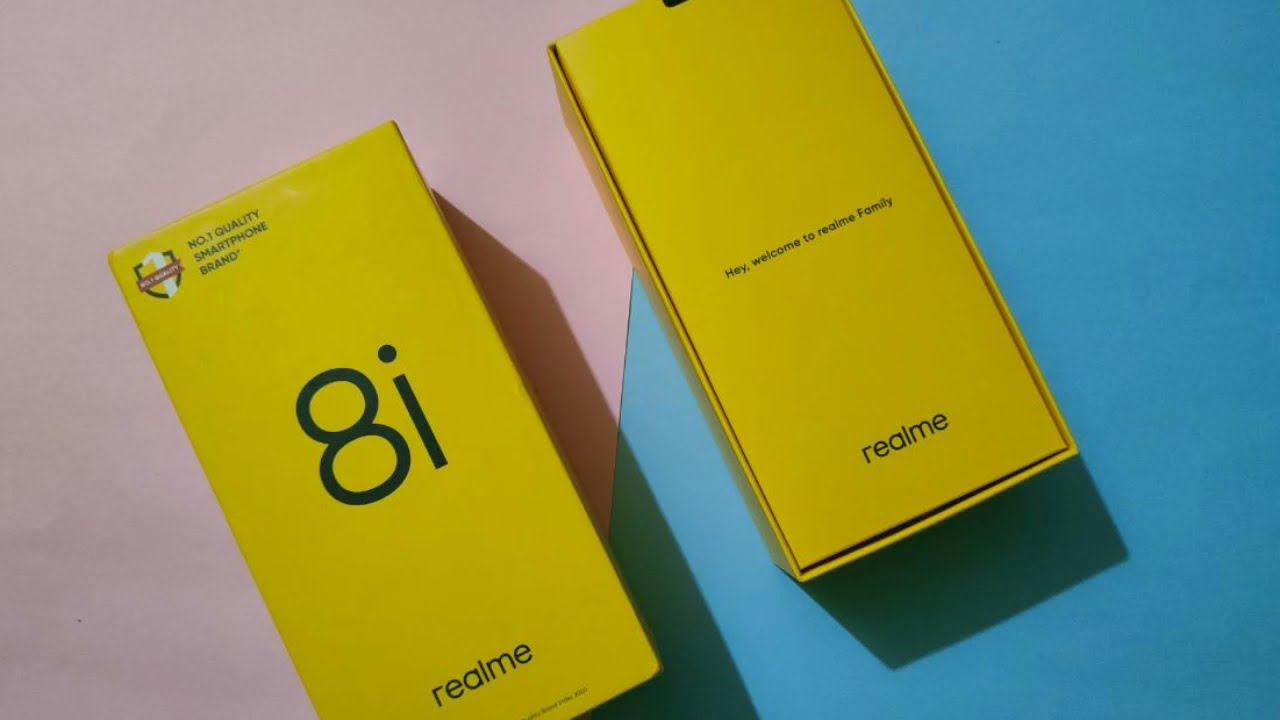The image showcases two rectangular yellow smartphone boxes set on a flat surface against a background that transitions from light purple on the left to medium blue on the right. The box on the left, tilted slightly upward to the left, displays its front side, featuring a number 1 icon with a shield at the top left, followed by the text "Number 1 Quality Smartphone Brand." The center of the box prominently displays "8i" in bold black letters, and at the bottom, "real me" is written in all lowercase, bold black letters. The box on the right shows the back side, with the words "Hey, welcome to the Real Me family" in small black print in the center, and "real me" again at the bottom in lowercase black letters. Both boxes cast subtle shadows, enhancing the overall composition of the image.